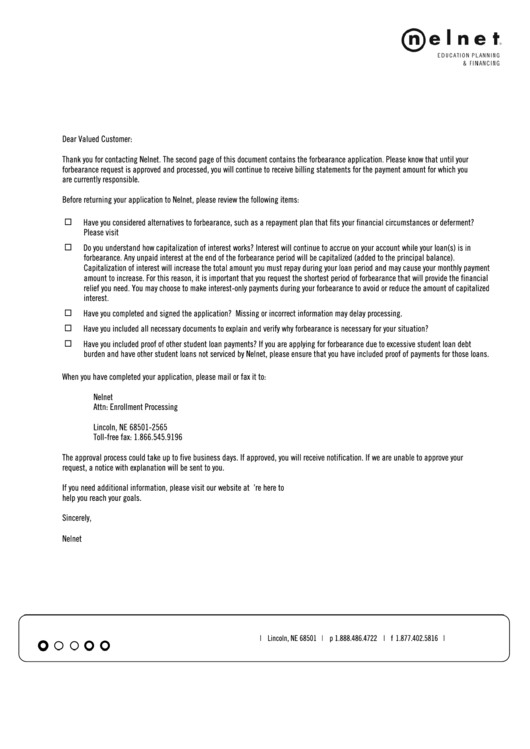The image depicts a letter, appearing either in the form of an email or an actual physical letter, addressed to a customer from Nelnet. The logo of Nelnet is positioned in the upper right-hand corner, characterized by a lowercase "n" encircled within a circle. The content intricately deals with education, planning, and finance.

The letter starts with a cordial greeting: "Dear Valued Customer," and proceeds to thank the recipient for reaching out to Nelnet. It informs the customer that the second page contains a forbearance application. A critical point mentioned is that until the forbearance request is approved and processed, the customer will continue to receive billing statements for the current payments they are responsible for. 

Before submitting the application back to Nelnet, the letter advises the customer to review the following checklist:
1. Consider alternatives.
2. Understand how capitalization of interest works.
3. Ensure the document is completed and signed.
4. Include all necessary documents.
5. Provide proof of other student loan payments.

Further instructions detail the process of mailing or faxing the completed application to Nelnet, Attention Enrollment Processing, in Lincoln, Nebraska, with the provided postal code 68501-2565. A toll-free fax number is supplied: 1.866.545.9196. The approval process is noted to take up to five days, during which notification will be given upon approval or a notice of explanation if the request is denied.

For additional information, the letter directs the customer to visit their website, though part of the URL appears to be incomplete due to missing characters. The message concludes with well-wishes for achieving the customer's goals, signed off "Sincerely, Nelnet."

The left margin of the letter contains five circles, with the first, fourth, and fifth circles in bold. The bottom section lists the address as Lincoln, Nebraska, 68501, alongside the phone and fax numbers again for convenience.